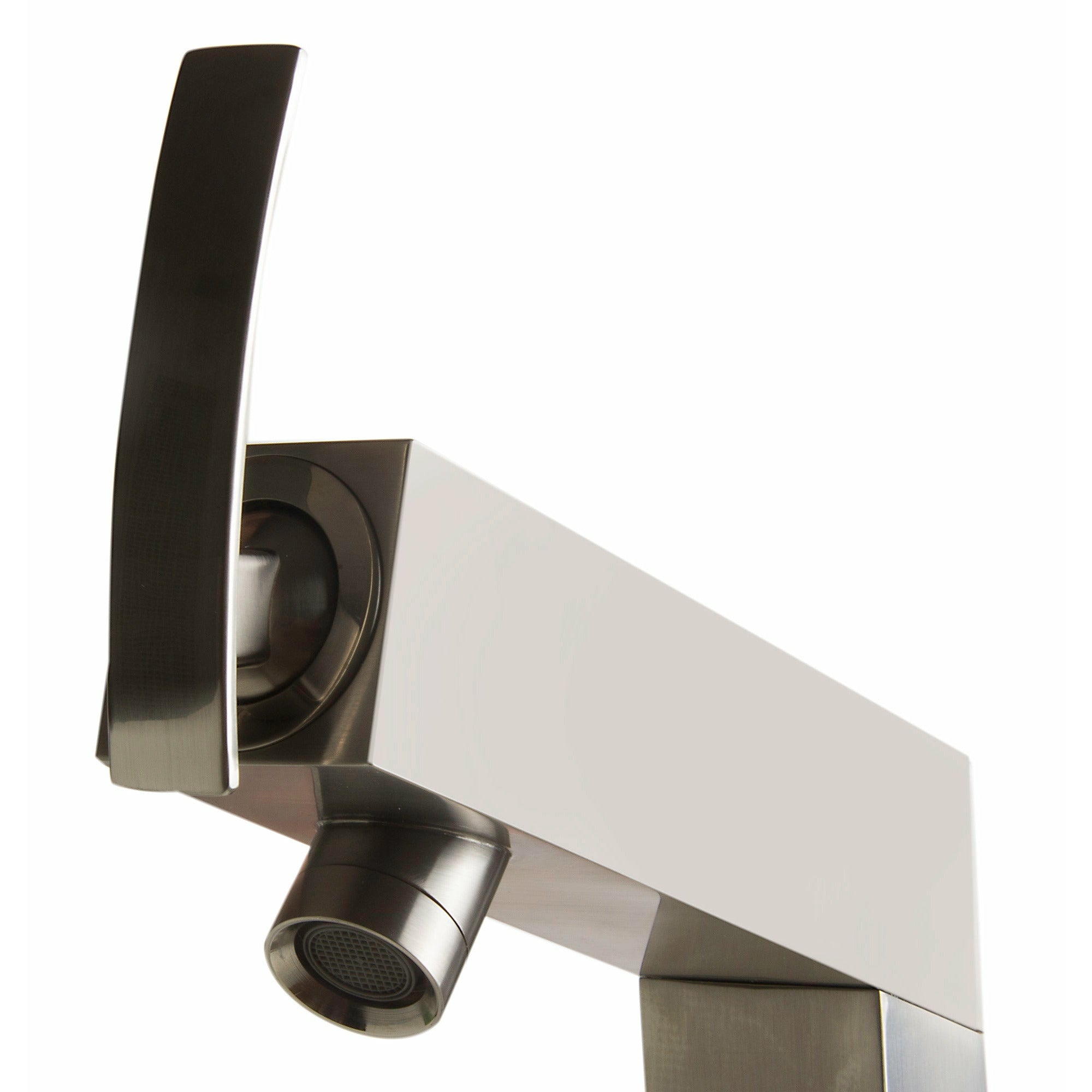The image showcases a security camera system set against a prominent white background. The camera itself is a long, rectangular metallic device with a sleek, modern design. Positioned at the left end of the rectangular unit is a large black lens encased within a circular metallic frame. This lens is partially obscured by a vertical metal bar that extends significantly beyond the camera's surface. At the bottom of the camera, there is a tube that features a black plastic grated area, possibly housing a speaker or microphone. The entire setup appears to be mounted on a stand or support structure, enhancing its functionality as part of a surveillance system.